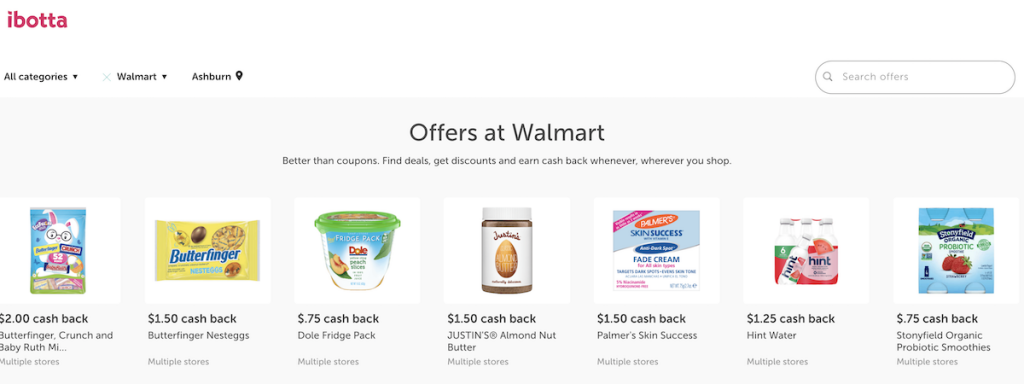Here is a detailed and clean caption:

"This image is a screenshot from the Ibotta website, which is indicated by the logo displayed in red in the upper left corner. Below the logo, there are navigation elements including 'All Categories' with a drop-down icon beside it, 'Walmart' with another drop-down icon next to it, and the location set to Ashburn with a location symbol to its right. On the far right side, near the top, there is a search bar labeled 'Search Offers' with a search button on its left.

Centered beneath the search bar, a promotional text reads: 'Offers at Walmart better than coupons. Find deals, get discounts, and earn cash back whenever and wherever you shop.' Listed prominently are the available cash-back offers, starting with:

1. Butterfinger Crunch
2. Butterfinger Nest Eggs
3. Dole Fridge Pack
4. Justin’s Almond Nut Butter
5. Palmer’s Skin Success
6. Hint Water
7. Stonyfield Organic Probiotic Smoothies

Each of these items is accompanied by a cash-back amount displayed in black above them."